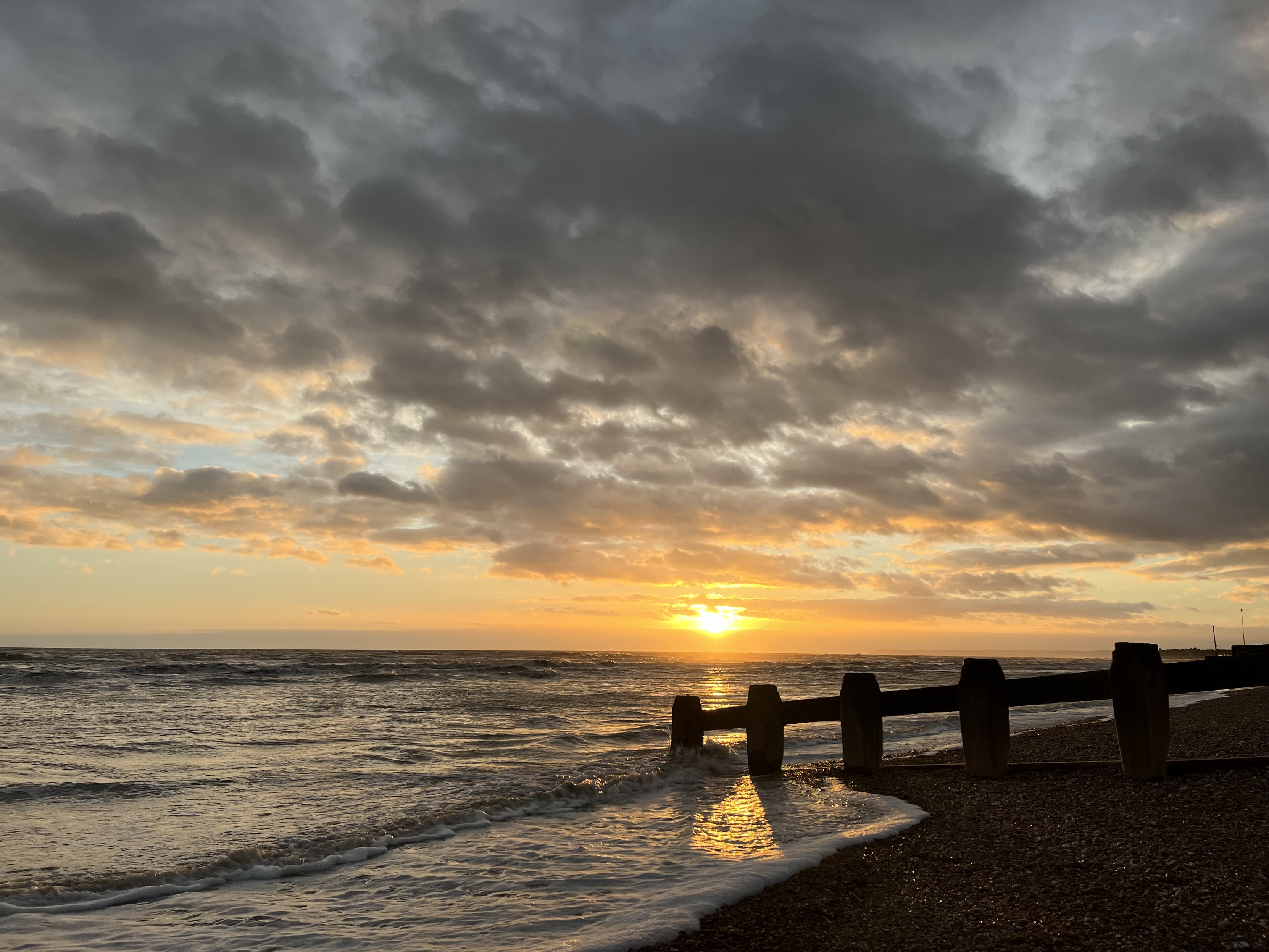The image captures a serene sunset over an ocean shoreline, with multifaceted details that create a rich visual tapestry. Dominating the scene is a bright orange sun centered near the horizon, casting a warm yellow and orange hue across a mostly overcast sky. The clouds vary from light to dark gray, interspersed with patches of clear sky, particularly to the left. The sun casts its vibrant light seamlessly across the tranquil yet slightly rough water, which transitions from a grayish blue to a foam-flecked shore where the waves gently break.

In the foreground, a wooden railing made from tree logs runs across the bottom part of the image, leading the eye along the beach to the right where the ocean meets the land. Emerging from the right side of the image is a silhouette of a pier, supported by five distinct posts and topped with a walkway, adding a structural element against the natural scene. Further in the distance, two antennas rise subtly into the sky. The beach itself is a mix of rocky and sandy textures, contrasting with the foamy waves ebbing at the shore. The composite effect of these elements forms a vivid and layered snapshot of a tranquil moment at the beach during sunset.